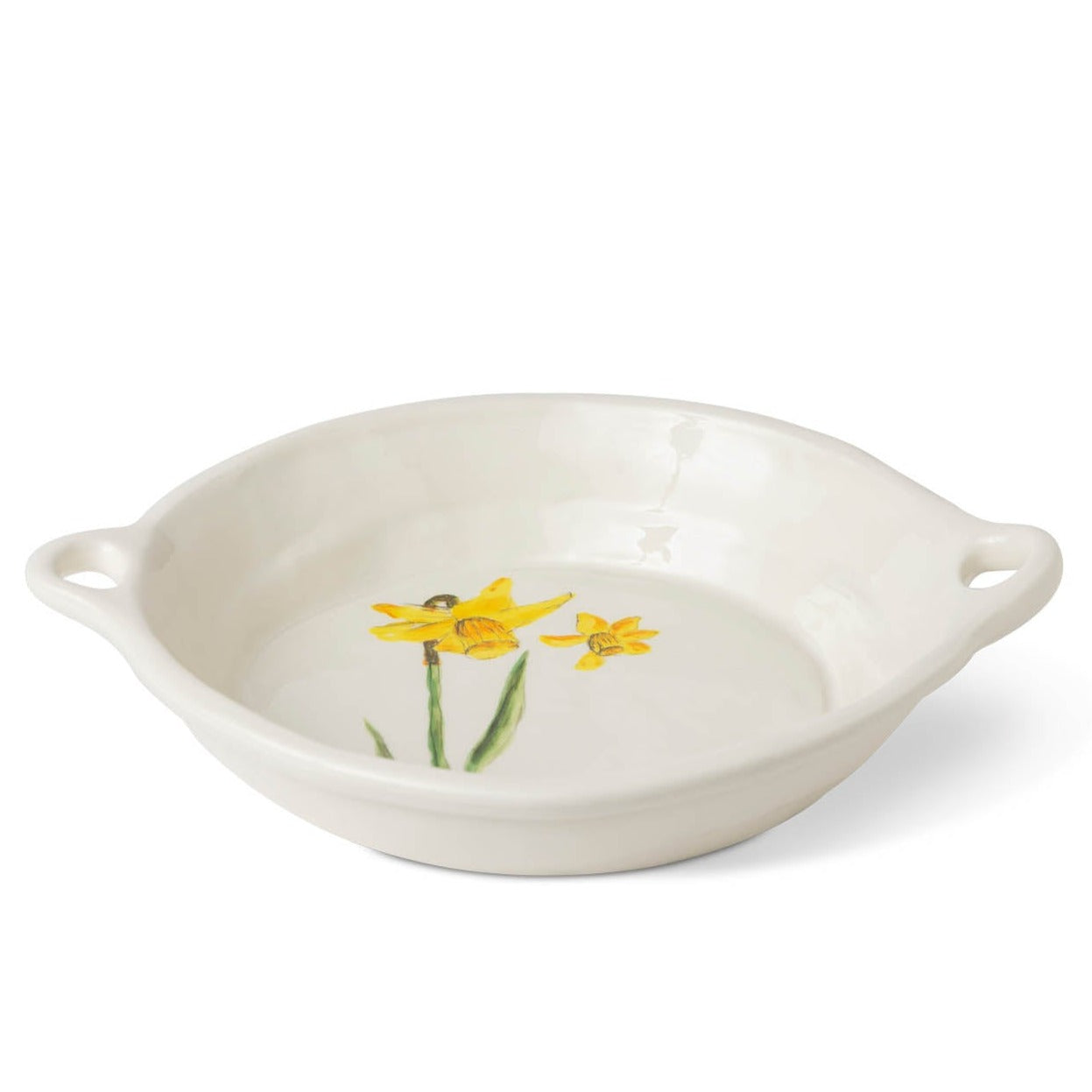This image is a detailed photograph of a horizontal, white ceramic serving dish with a handle on either side. The dish has a grayish tint and sits on a perfectly white background. In the center of the dish, there is an artistic depiction of two yellow daffodil flowers with green stems, along with a partially hidden third green leaf at the bottom. The daffodils notably stand out against the light background, enhancing their visibility and adding a touch of elegance to the otherwise simple design. The dish is shallow and versatile, suitable for serving vegetables or similar types of food.